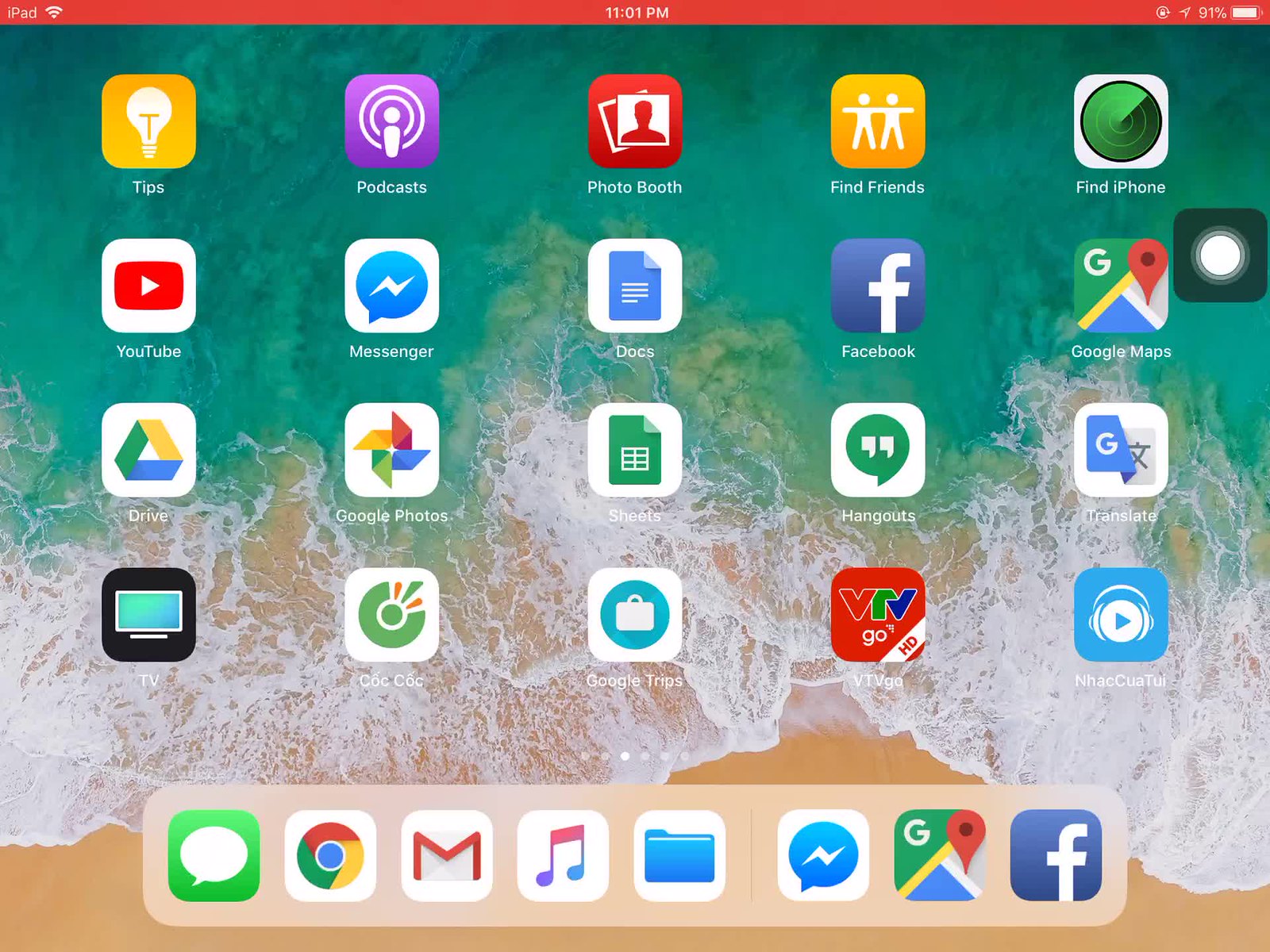The image showcases the home screen of a phone or tablet, featuring a vibrant, beach-themed background. The backdrop captures a serene shoreline with clear, greenish-blue water gently meeting the sandy beach which exhibits various shades of brown.

The home screen is populated with a variety of apps:
- A yellow "Tips" app.
- A purple "Podcast" app.
- A red "Photo Booth" app.
- A yellow "Find Friends" app.
- A green "Find iPhone" app, previously referred to as "Planet."
- A red and white "YouTube" app.
- A blue and white "Messenger" app.
- A blue and white "Docs" app.
- A blue and white "Facebook" app.
- A "Google Maps" app, identifiable by its green, blue, and white icon with a red location pin.
- At the bottom of the screen, there's the "Google Photos" app.

This detailed array of applications, set against the calming and picturesque beach background, suggests a well-organized and visually appealing digital home space.